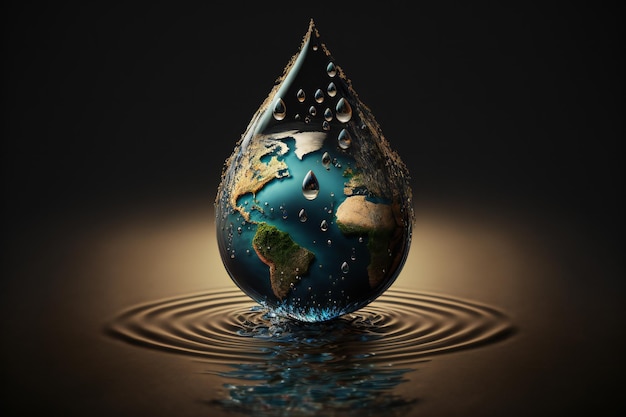This digital render, featuring an intricate and unique artistic concept, showcases a photorealistic illustration of a single large water droplet suspended just above a rippling, dark golden-brown surface. The background remains starkly black, emphasizing the central focus. 

Embedded within this large droplet is a detailed, three-dimensional depiction of planet Earth, highlighting continents such as North America, South America, Africa, Europe, and Asia in hues of blue, green, tan, and white. Surrounding the main droplet are smaller droplets, suggesting condensation running down its surface. Reflections of the droplet and Earth are visible in the water below, contributing to the illusion of depth and dimensionality. The droplet's contact with the surface generates concentric ripple effects extending outwards, enhancing the dynamic and immersive quality of the image.